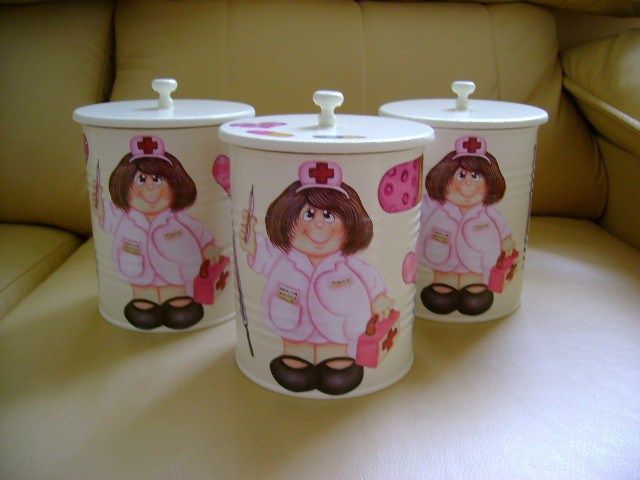This photograph captures three identical white canisters, each adorned with an illustration of a cartoon nurse. The nurse depicted is female, with short brown hair, dressed in a pink uniform that includes a coat and a hat with a red cross emblem. She is holding a syringe in one hand and a pink medical box with a red cross in the other. The canisters are characterized by circular lids with knobs on top and are all placed on a light brown sofa. The nurse illustration further includes black shoes, and she appears big and fluffy. The image is taken in a landscape orientation.